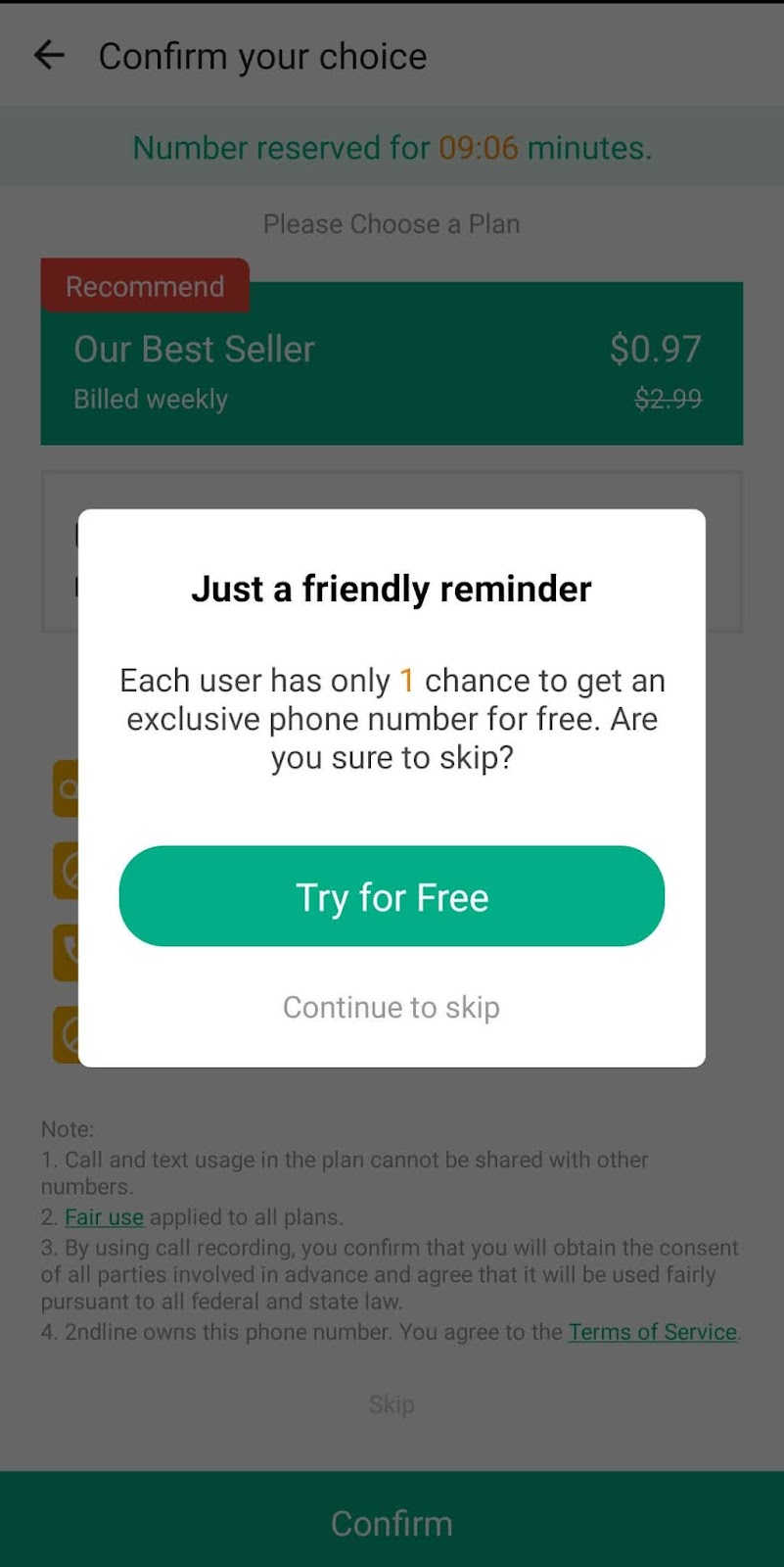The image is a screenshot of an application interface with a pop-up box prominently displayed. The background of the application is dimmed to emphasize the pop-up box, although the faded elements are still partially visible. The pop-up box itself is white, featuring black text that reads, "Just a friendly reminder: Each user has one chance to get an exclusive phone number for free. Are you sure you want to skip?" Beneath this text, there is a green button labeled "Try for Free" and an adjacent link with the text "Continue to Skip."

The semi-transparent background reveals additional text and interface elements. At the top, there is a back arrow with text that reads "Confirm Your Choice." A timer indicates that the number is reserved for "9.6 minutes." Below the timer is a prompt to "Please choose a plan."

A red banner labeled "Recommended" highlights the best-selling plan, which is priced at 97 cents but billed weekly. The regular price of $2.99 is crossed out to indicate a discount.

Although the pop-up box obstructs much of the application's interface, some yellow buttons are visible at the bottom. Additionally, there is a green button labeled "Confirm" at the bottom of the pop-up box.